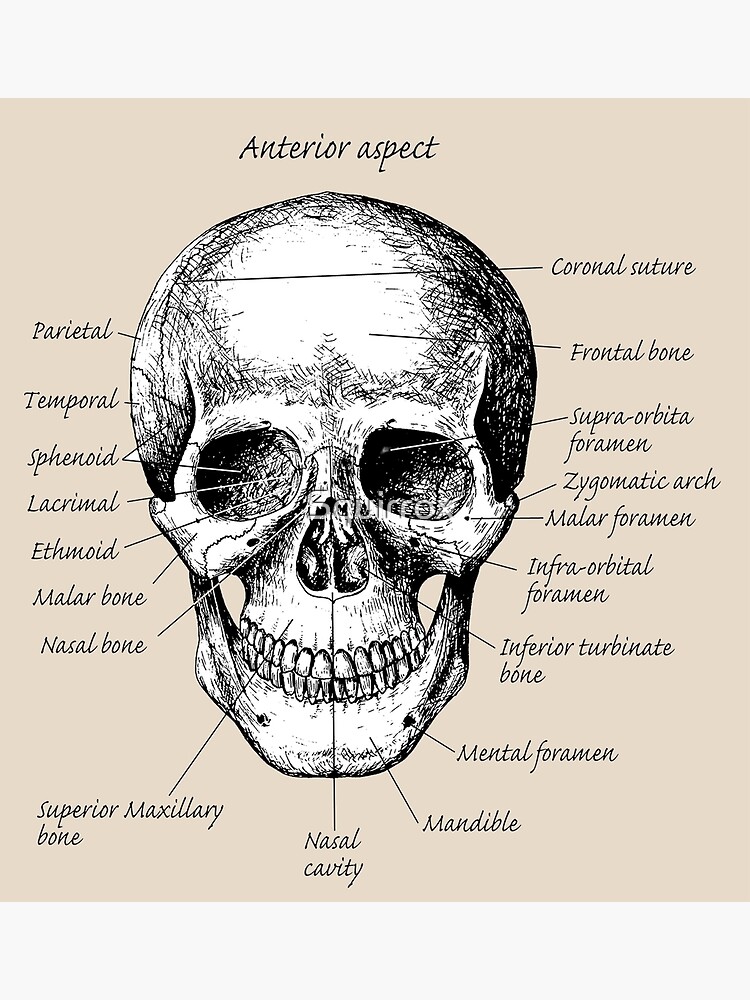This scientific drawing depicts an anterior aspect view of a human skull, rendered in detailed black and white pencil shading. The skull is prominently labeled with anatomical and scientific terms in gray script, all accurately identifying various sections and functions. The labeling follows a loop from the right-hand side, detailing parts such as the coronal suture, frontal bone, supraorbital foramen, zygomatic arch, malar foramen, infraorbital foramen, inferior turbinate bone, mental foramen, mandible, nasal cavity, superior maxillary bone, nasal bone, malar bone, ethmoid, lacrimal, sphenoid, temporal, and parietal bones. The backdrop of the image is a subtle taupe or sepia color, enhancing the clarity of the white skull shaded in gray. There's a faint copyright overlay that doesn't obscure the intricate details. The image serves as an educational, medical diagram, meticulously outlining the complex structure and various sections of the human skull.